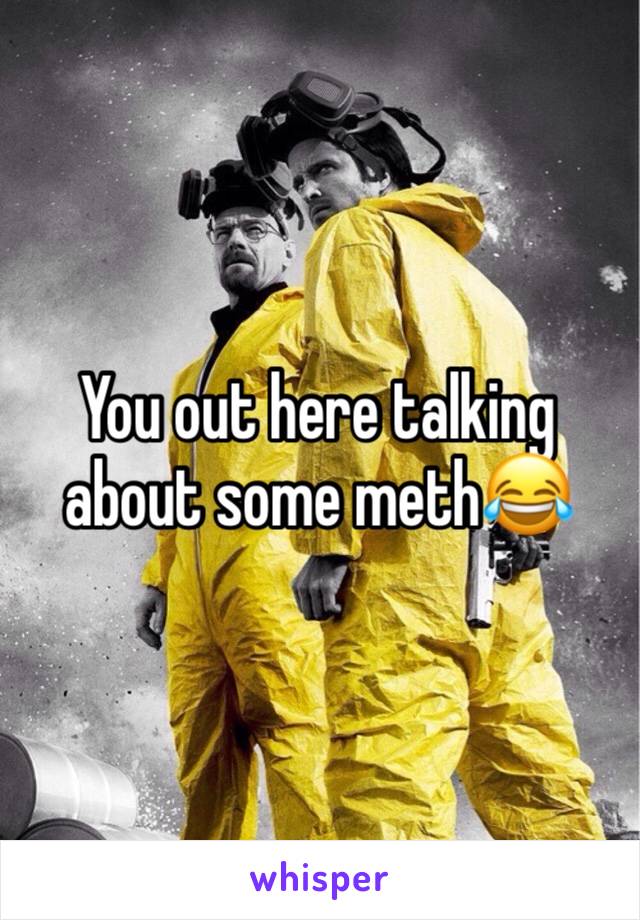In this highly detailed, black-and-white photograph with spot color added, two men, iconic characters from the TV series Breaking Bad portrayed by Bryan Cranston and Aaron Paul, are captured in a tense, atmospheric scene. The image, set against a stormy background highlighted with sparkles, showcases the men donning bright yellow hazmat suits and gas masks. Bryan Cranston, almost facing the camera, is positioned slightly behind and to the left of Aaron Paul, who faces away from the viewer but looks back over his shoulder while discretely holding a silver pistol behind his back. To the left of the men, on the ground, are two barrels, suggesting the setting involves hazardous materials. Overlaying this striking scene is text in white font with a black outline, reading, "You out here talking about some M.E.T.H.," accompanied by a crying smiley face emoji. Below the image, in dark purple, lowercase script, is the word "whisper," anchoring the caption with a stylistic touch of typo-graphical realism.